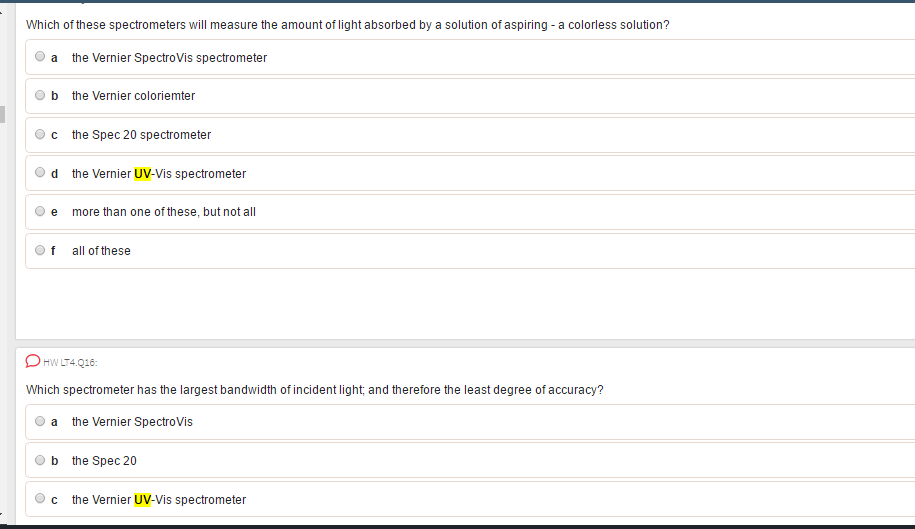The image depicts a question examining knowledge of various spectrometers and their functions. The background is predominantly white with a thin black border at the top and bottom. Central to the image is a rectangular segment, oriented horizontally. 

At the top of this rectangle, there is a text prompt: "Which of these spectrometers will measure the amount of light absorbed by a solution of aspirin - a colorless solution?" Below this question, there are multiple-choice options, labeled A through F, each with a circular bubble next to it for selection. The options are as follows:
A) Verner Spectrometer
B) Verner Colorimeter
C) Spec 20 Spectrometer
D) Verner UV-Vis Spectrometer (Highlighted in yellow)
E) More than one of these but not all
F) All of these

Below this first multiple-choice question, there is an additional query: "Which spectrometer has the largest bandwidth of incident light and therefore the least degree of accuracy?" with the reference "HWLT4.Q16." The answer choices for this question, labeled A through C, are:
A) Verner Spectrometer
B) Spec 20 Spectrometer
C) Verner UV-Vis Spectrometer (Highlighted in yellow)

None of the selection bubbles for the answers have been filled in.